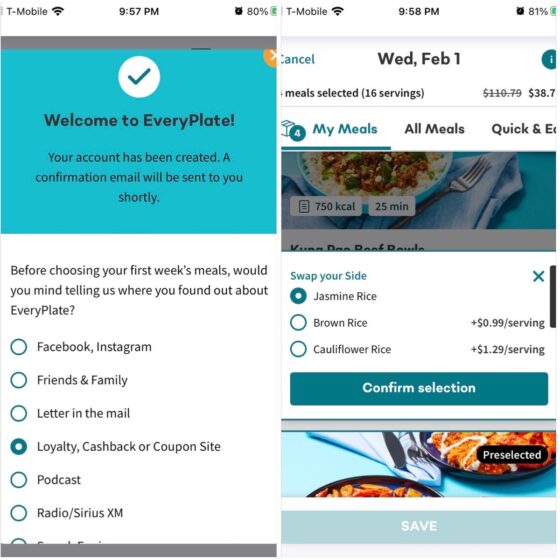The image is composed of two screenshots from likely the same app or mobile website, showcasing different stages of user interaction. 

In the left screenshot, positioned in the center, there is a welcome message from EveryPlate stating, "Welcome to EveryPlate! Your account has been created. A confirmation email will be sent to you shortly." Below this, the user is prompted to share how they discovered EveryPlate, with multiple options provided: Facebook, Instagram, friends and family, letter in the mail, loyalty cashback or coupon site, podcast, and radio/SiriusXM. The option "loyalty cashback or coupon site" is highlighted in blue, indicating it has been selected.

The right screenshot displays a page labeled "Wednesday, February 1st" at the top, under the "My Meals" tab. Below this heading, it prompts the user to "Swap your side," offering three choices: Jasmine Rice, Brown Rice, or Cauliflower Rice. Next to "Brown Rice," there is a note indicating an additional cost of $0.99 per serving, while "Cauliflower Rice" is listed with an extra charge of $1.29 per serving. At the bottom, there is a teal-colored button labeled "Confirm Selection."